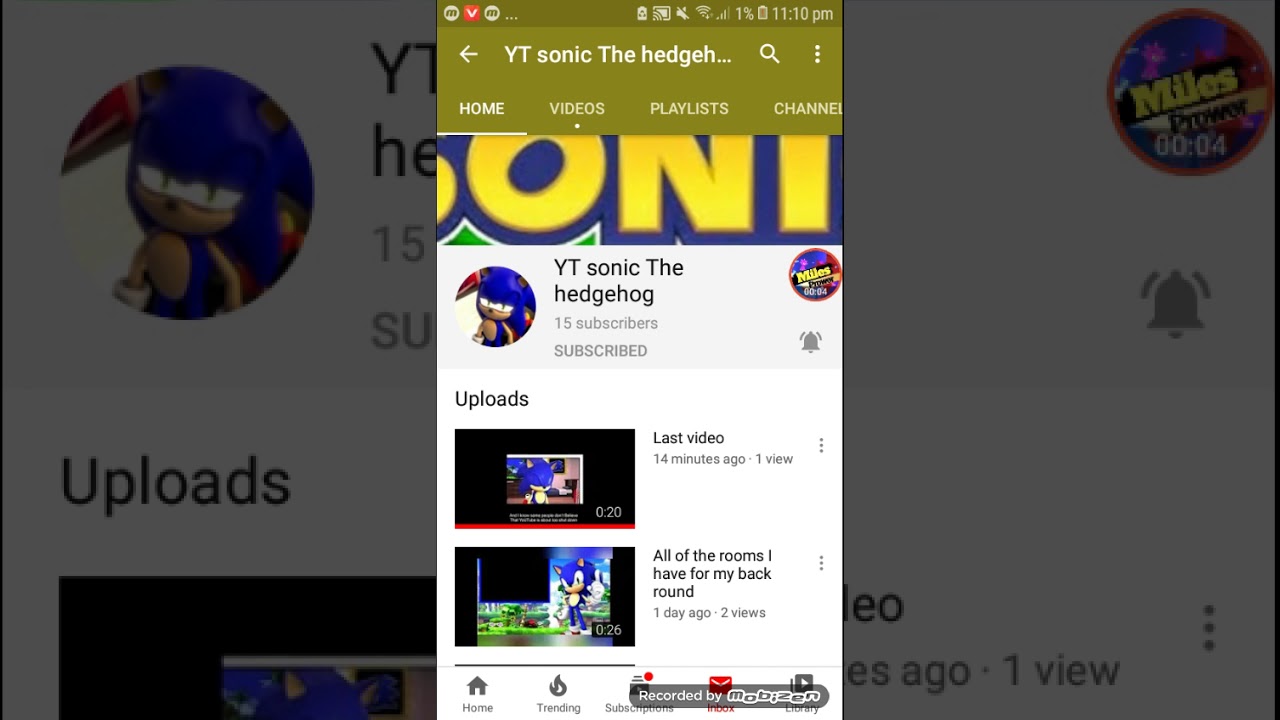Here's a detailed and cleaned-up description of the image in the screenshot:

---

This image is a screenshot of a YouTube channel called "YT Sonic the Hedgehog." The channel features an image of Sonic the Hedgehog as its profile picture and currently has 15 subscribers, with the viewer being subscribed to the channel. The channel's primary tabs include Home, Videos, Playlists, and Channels.

The screenshot was taken at 11:10 PM with the device's battery life critically low at 1%, activating the battery saver mode. The content is being viewed on a TV or another larger screen, possibly through a streaming device.

Two videos are highlighted in the screenshot:

1. The first video, titled "The Last Video," was uploaded 14 minutes ago and features an image of Sonic the Hedgehog on a screen.
2. The second video, titled "All of My Rooms I Have from My Background," was uploaded one day ago and has received two views. This 26-second video showcases Sonic the Hedgehog in a colorful environment.

Navigation icons for Home, Trending, Subscriptions, Inbox, and Library are visible at the bottom of the screen. There is a "Recorded by Mobizen" watermark indicating the use of screen recording software. Additionally, the screenshot mentions "Miles 'Tails' Prower," hinting at the presence of Sonic's famous sidekick, although this context is unclear.

Overall, the screenshot captures essential information about the "YT Sonic the Hedgehog" YouTube channel, its subscriber count, recent uploads, and viewing conditions.